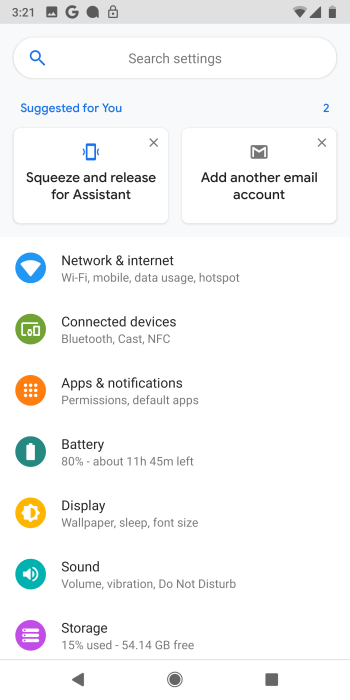Screenshot of a smartphone display at 3:21 PM, showcasing various settings. The screen features a search bar at the top with a blue magnifying glass icon to the left labeled “Search settings.” Beneath the search bar, there are three suggested options: "Suggested for you," "Squeeze and release for assistance," and "Add another email account."

The settings menu displays numerous categories:

1. **Network & Internet**: Options for Wi-Fi, mobile data usage, and hotspots.
2. **Connected Devices**: Includes settings for Bluetooth, Cast, and NFC.
3. **Apps & Notifications**: Covers app permissions and default apps settings.
4. **Battery**: Displays 80% battery life with an estimated 11 hours and 45 minutes remaining.
5. **Display**: Settings for wallpaper, sleep mode, and font size.
6. **Sound**: Controls for volume, vibration, and Do Not Disturb mode.
7. **Storage**: Shows 15% storage used, with 54.14 GB of 64 GB available.

The user is navigating these settings to customize their device’s functionalities and preferences.